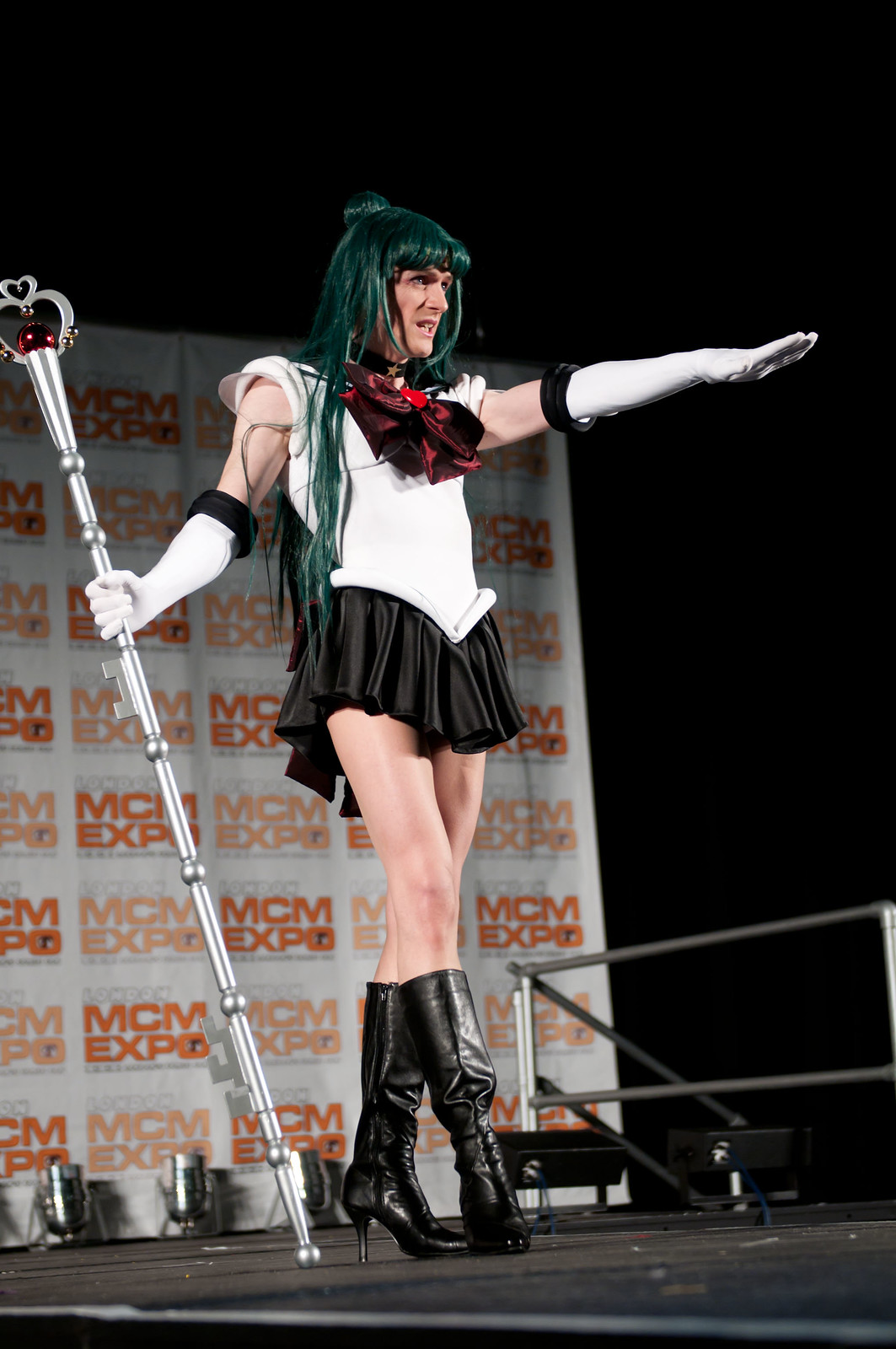In this detailed indoor photograph, a man dressed in a magical girl cosplay outfit, reminiscent of Sailor Moon, stands on a black stage in what appears to be a conference or hotel room. He wears a long green wig that cascades over his shoulders, and a costume consisting of a sleeveless white top connected to a very short black skirt that falls well above his knees. His ensemble is completed with black high-heeled boots that reach just below his knees and long, white elbow-length gloves adorned with black bands. In his left arm, he carries a staff topped with a crown-like ornament, which adds a regal touch to his appearance. The man gazes off into the distance, striking a pose that accentuates the theatricality of his attire. The backdrop features a prominent orange sign that reads "MCM Expo," accompanied by a railing and spotlights, which highlight the event's grandeur.